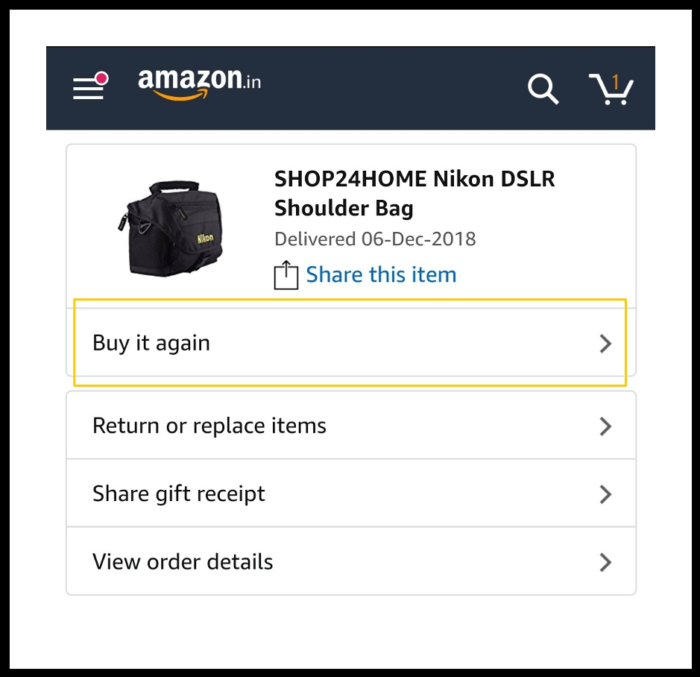The image displays an Amazon order summary against a bright white background, framed with a thin black border. At the top of the image, the Amazon header is visible, featuring a menu button on the left with a red notification circle. Positioned centrally is the Amazon.in logo, complete with the iconic yellow arrow pointing from 'A' to 'Z', symbolizing the variety of products available. To the right of the logo, a white magnifying glass icon represents the search function, followed by a white shopping cart icon showing one item inside.

Beneath the header, the purchased item is detailed: a "Shop 24 Home Nikon DSLR Shoulder Bag," which was delivered on December 6, 2018. Several options are available below the item description, including sharing the item, buying it again (highlighted with a gold box), returning or replacing items, sharing a gift receipt, and viewing order details.